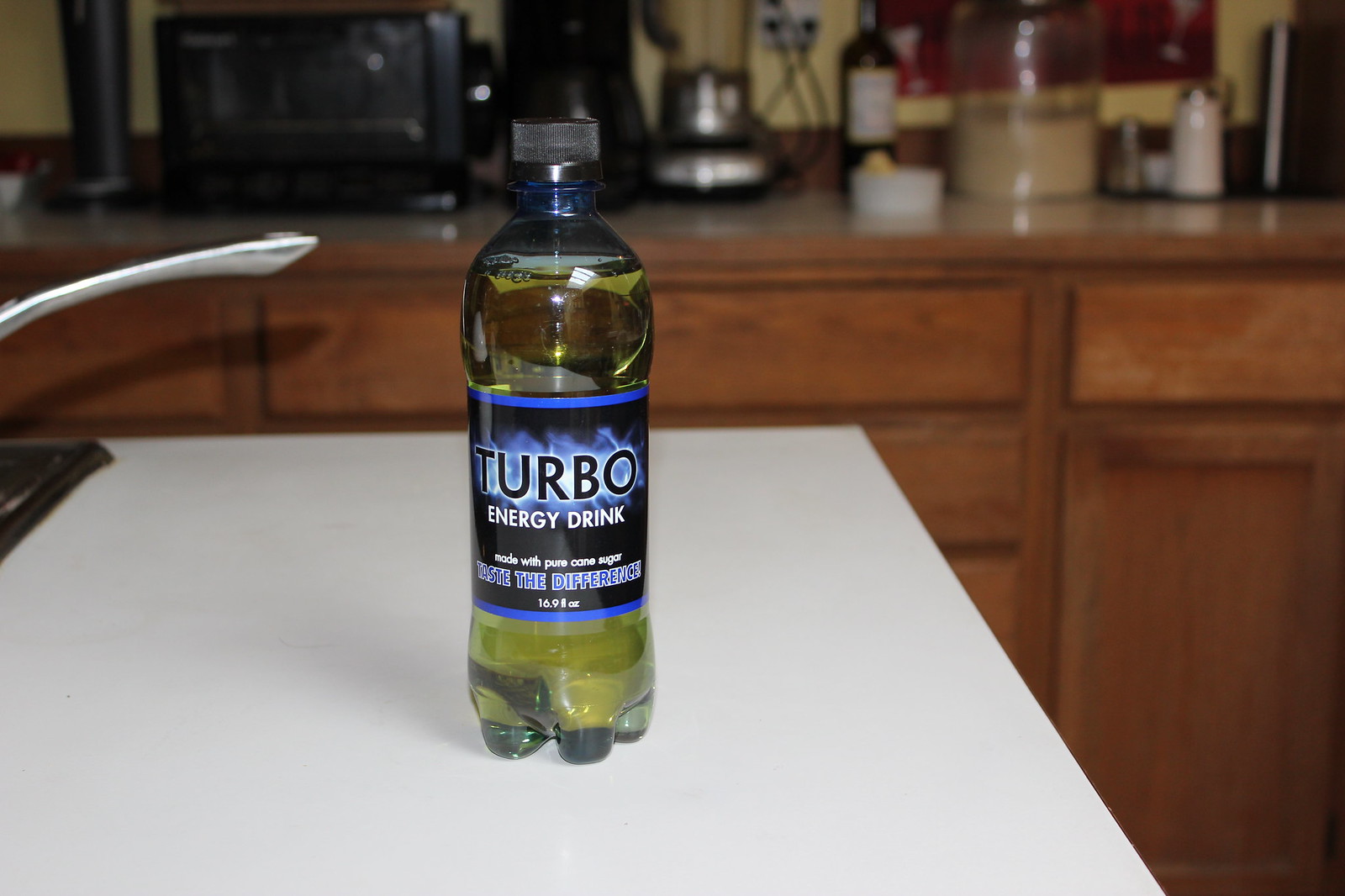In this close-up photograph of a kitchen scene, the primary focus is a cylindrical plastic bottle of Turbo Energy Drink, prominently displayed on a white countertop. The bottle contains a yellowish-green liquid and features a detailed label with "Turbo Energy Drink" written in black and white text, along with the phrases "Taste the Difference," "16.9 fluid ounces," and "Made with pure cane sugar." The bottle is capped with a black twist top.

Surrounding the bottle, a variety of kitchen appliances and items are visible against the backdrop of dark brown lower cabinets and a tan countertop. To the left, slightly blurred, is a stove with a silver handle. On the countertop, there is a black microwave, a silver blender with a glass top, a glass jar containing a brown substance, and a cylindrical white salt shaker with a silver top. The image captures a contemporary kitchen setting, though some details are slightly obscured due to the depth of field.